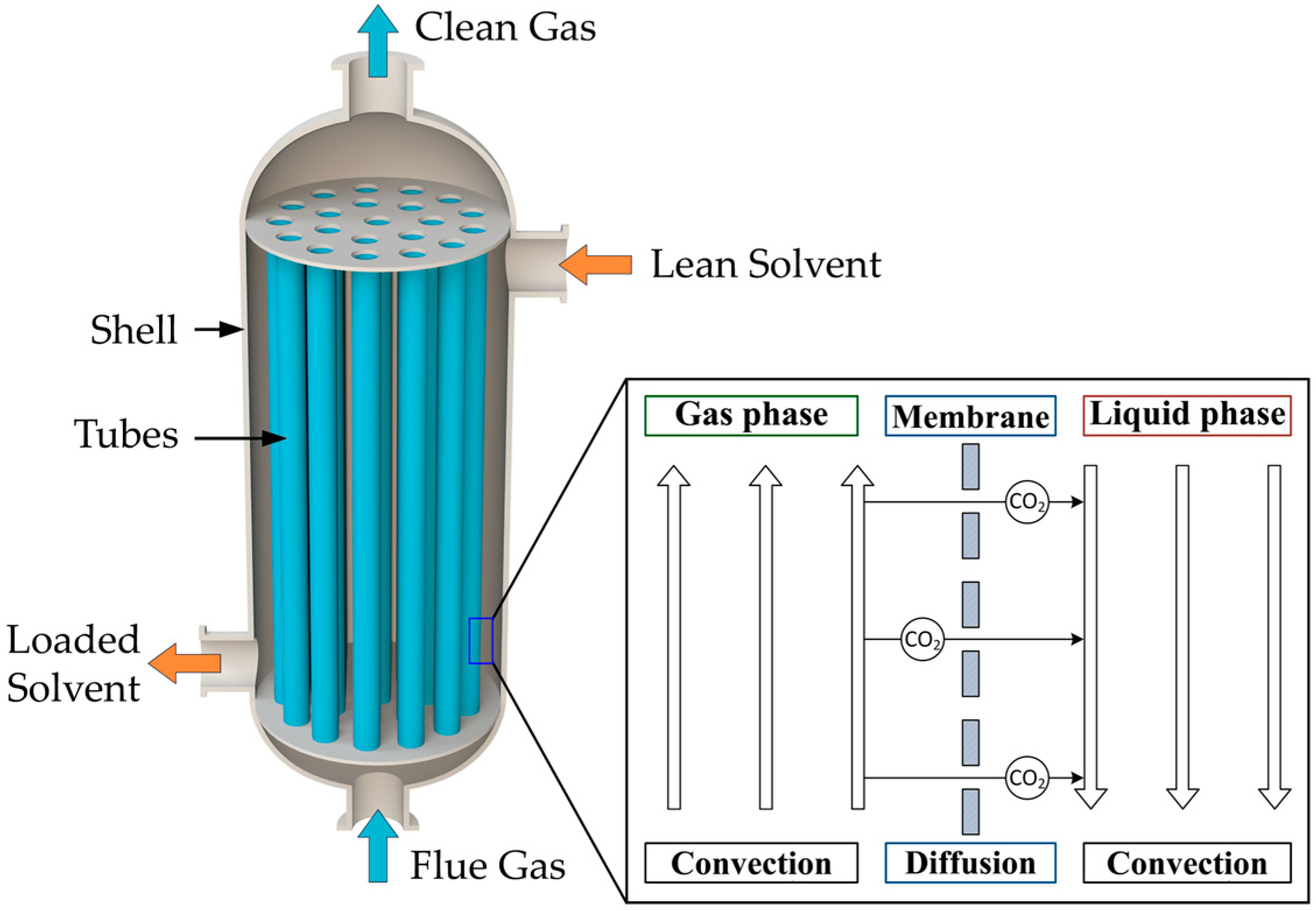The image depicts a detailed technical illustration of a gas system against a featureless white background. Dominating the left part of the frame is a cylindrical object with an exposed inner section, revealing vertical, neon blue, dowel-shaped tubes. These tubes are capped at both ends by flat, circular gray metal plates. Blue dots mark the connection points at the top plate, and above this assembly is a cutaway view of a metal dome, leading to a tube labeled "clean gas" exiting upwards.

Further details include a tube labeled "lean solvent" entering the cylinder from the right, an intake tube at the bottom marked "flue gas," and an outtake tube on the lower left labeled "loaded solvent." The exterior shell surrounding the blue tubes has been partially cut away for clarity, and these tubes as well as the shell itself are clearly labeled.

To the right of the cylinder, a technical flowchart visualizes the system's functioning. It features red, blue, and green boxes labeled "liquid phase," "membrane," and "gas phase" respectively, alongside directional arrows and annotations. This diagram includes terms such as "convection" and "diffusion," with lines marked "CO2," illustrating the processes involved in the gas system.